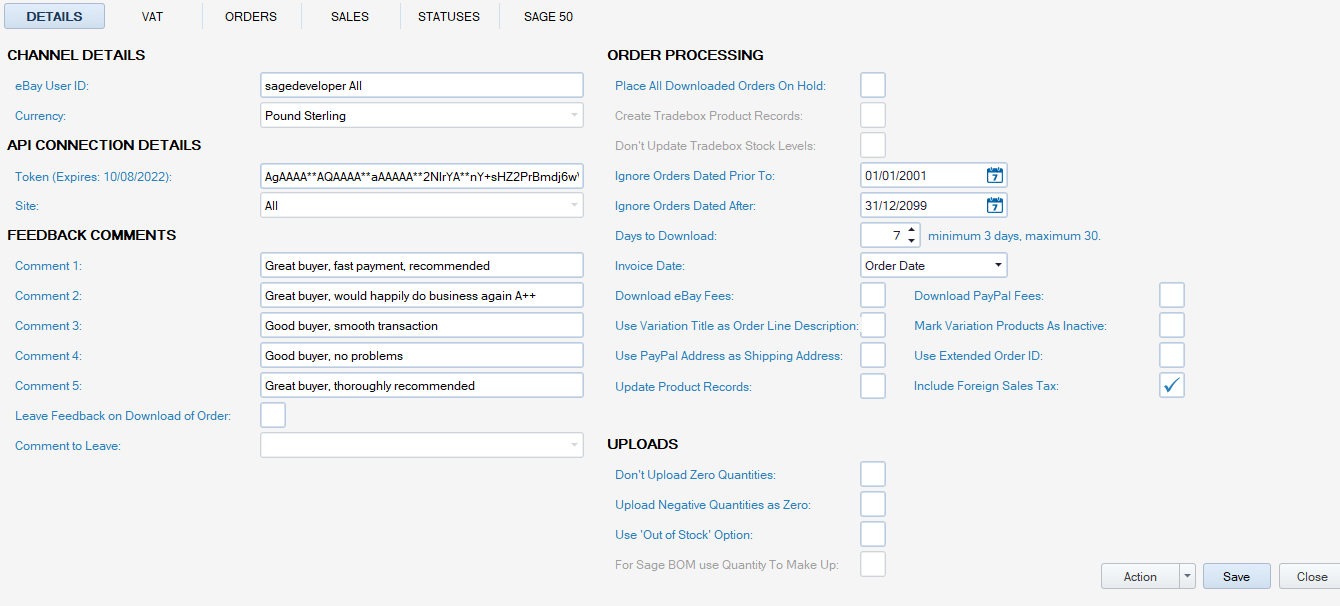Screenshot of a comprehensive eBay e-commerce accounting form used for digital products or dropshipping. The form is presented on a light gray background with blue text for input fields and all caps for titles. The screen is labeled "DETAILS."

Starting with the "CHANNEL DETAILS" section, the form indicates:

- **eBay User ID:** Sage Developer All
- **Currency:** Pound Sterling (£)
- **API Connection Details:**
  - Token expiration: October 2022
  - Site: All
- **Feedback Comments:** 
  - 5 comments listed as:
    - Great buyer
    - Great buyer
    - Good buyer
    - Good buyer
    - Great buyer

Additional controls include:

- **Order Processing:**
  - Place all downloaded orders on hold: Not checked
  - Ignore orders dated prior to January 1, 2001
  - Ignore orders dated after December 2099

The form displays options for uploads, downloads, actions, saving, and closing. At the very top, the available menu options include VAT, Orders, Details, Statuses, and Sage 50.